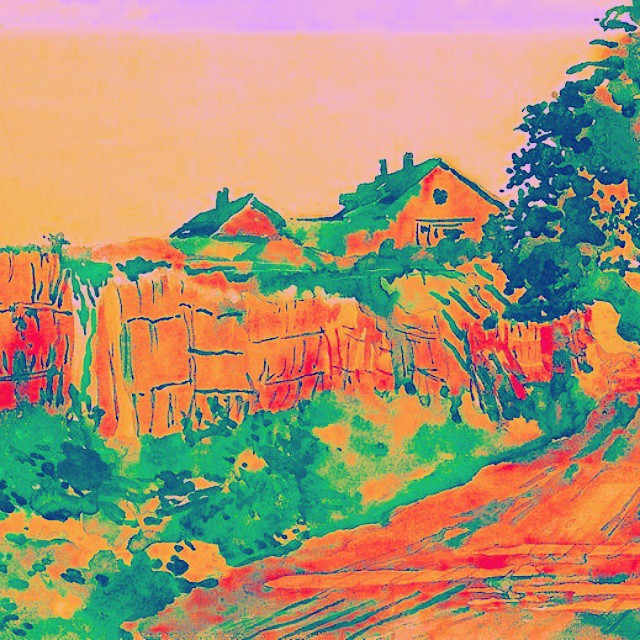This vibrant painting uses an array of bright colors to depict a serene country scene. The composition is rich with oranges, greens, golds, and reds, creating a lively yet harmonious palette. The viewpoint is set from a country road, looking towards a gentle grassy incline. At the top of this incline stands a fence, strikingly painted in shades of orange and red, with vivid blue horizontal lines mimicking seams that hold the structure together.

Beyond the fence, the greenery continues, leading the eye slightly up the road where the side of a large tree becomes visible. The tree's leaves are an artistic blend of blues and greens, adding depth and texture. Adjacent to this, a house emerges, its walls painted a warm orange while the roof features a mix of blues and greens, indicating a shingled texture. The house has two chimneys, suggesting a cozy and functional residence.

A covered walkway extends from the main house to a smaller structure, which shares the same colorful roof but is painted in a brighter, orangish-red hue. This secondary building adds an additional layer of interest and balance to the composition. Overall, the use of bold, contrasting colors and detailed elements gives this painting a dynamic and picturesque quality, capturing the charm of rural life.